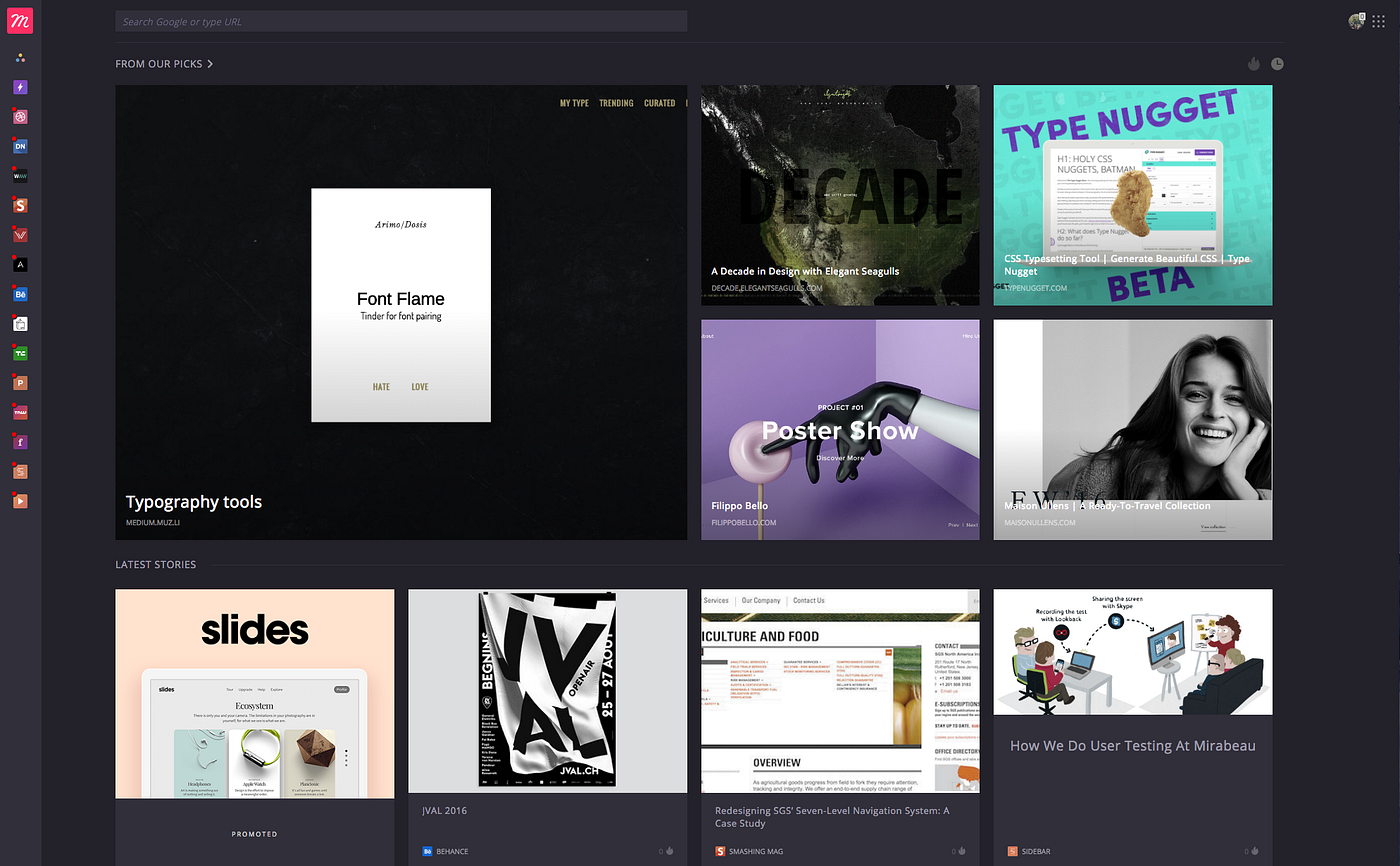The image is a rectangular layout with the longer side extending horizontally. The background is entirely black. On the left side, there is a narrow vertical column featuring various icons. The icon at the very top is a red box with the letter "M" inside it. The other icons in the column vary in symbols and colors, though their details are indistinguishable.

To the right of this column, near the top, there is a search box. Further to the right, in the top corner, are two additional icons whose details are not clear. 

The main section of the image contains several distinct sections. At the top, there is a large black rectangle with an inset white box that reads "Font Flame." There is additional text within this box, but it is too small to decipher.

Below, there is a larger black rectangle labeled "Typography Tools." Surrounding this central black box are eight smaller boxes. Starting from the bottom left and moving to the right, one box is labeled "Slides," and another box to its right contains a black and white flag-like symbol. Another box is labeled "Agricultural and Food." The remaining boxes have various labels and symbols, but their specifics are not mentioned.